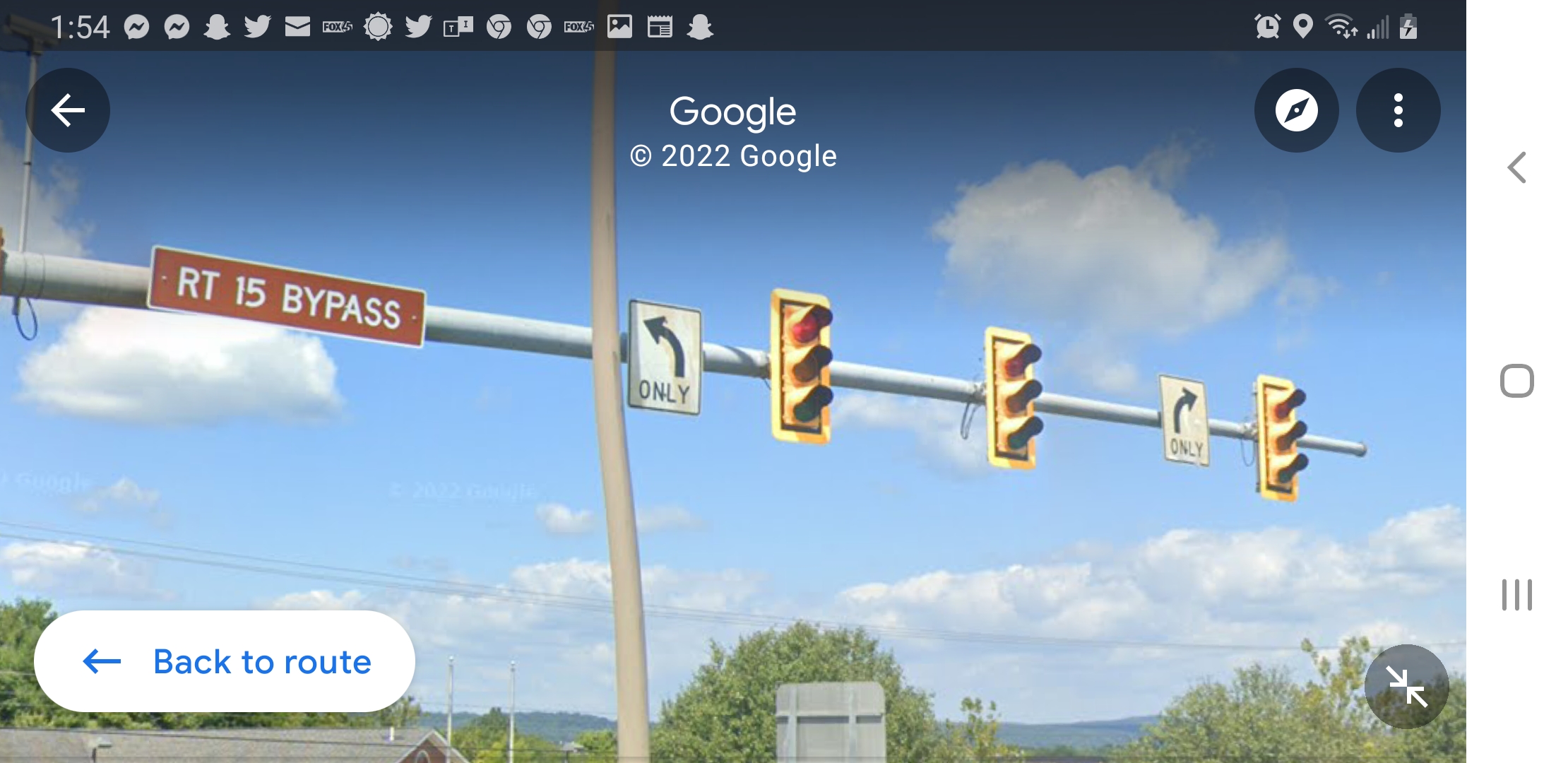The image depicts a screenshot from a Google Maps view. In the top left corner, the time display reads 1:54, surrounded by various cell phone icons on a black background. Directly below, a white arrow enclosed in a black circle directs left, adjacent to the Google logo marked as "2002 Google," with two additional icons to its right.

In the central part of the image, a series of vertical traffic lights, housed in yellow rectangular boxes, display red, yellow, and green lights. These traffic lights are mounted on intersecting gray and brown poles. Nearby, on the left side of the image, a brown sign with white text indicates "RT-15 Bypass."

Towards the bottom left, there's blue text reading "Back to route," accompanied by a blue arrow. The lower section of the image is dominated by lush green trees, with a light blue sky and scattered clouds above them, enveloping the scene in a serene, open-air setting.